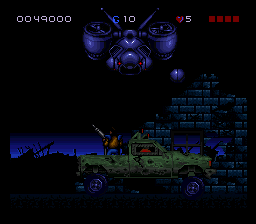This square screenshot, captured from a video game, depicts a nighttime scene filled with ominous elements and intricate details. Dominating the center is a green pickup truck navigating a pitch-black road, with its path partially obstructed by a fragmented brick wall. Above, white writing displays vital game statistics, accompanied by a heart icon and several red symbols. Shadows cast by trees loom in the background against a starkly contrasting blue horizon, under an impenetrably black sky. Hovering ominously in the sky is a monstrous, robot-like figure, bathed in purple with striking white and red accents. Adding to the scene's tension, a person clad in a yellow vest stands in the truck bed, aiming a gun skyward.